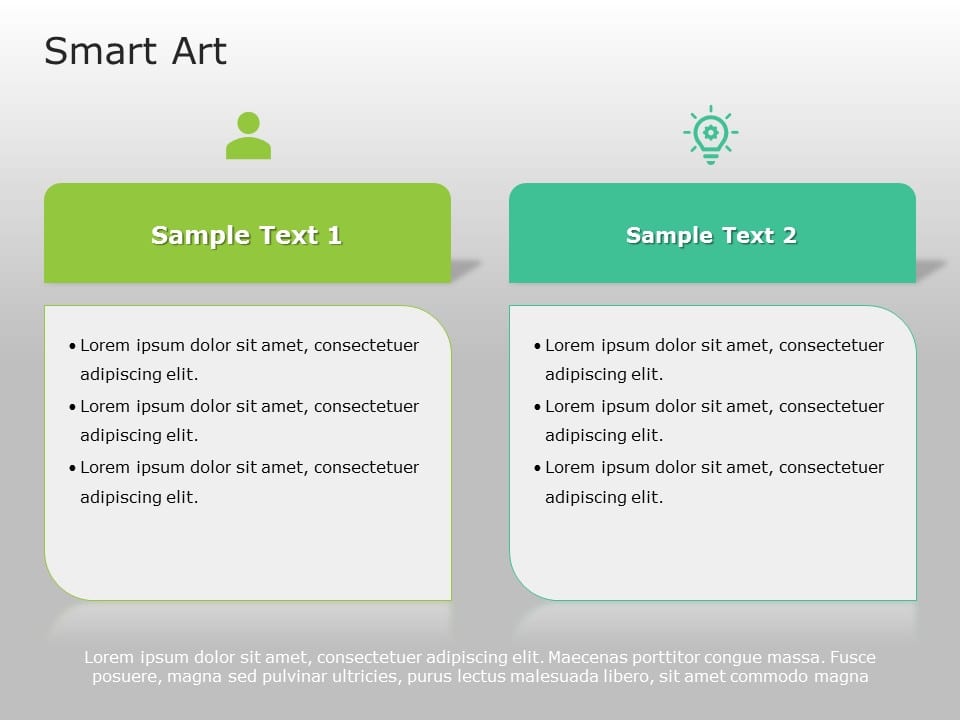The image features what appears to be a web page or infographic template titled "Smart Art" in black text at the top left. The layout consists of two main columns. The left column has a simplified logo of a person, depicted as a round head and semi-circular body, above a green card with the white text "Sample Text One." Below this is a white card containing three bulleted paragraphs of placeholder text, often referred to as Lorem Ipsum. 

The right column mirrors the structure of the left but begins with a stylized light bulb icon in a greenish-turquoise color above a similarly colored card with the white text "Sample Text Two." Another white card is situated below with additional Lorem Ipsum text across two rows. The overall background is gray, providing a neutral backdrop for these elements.